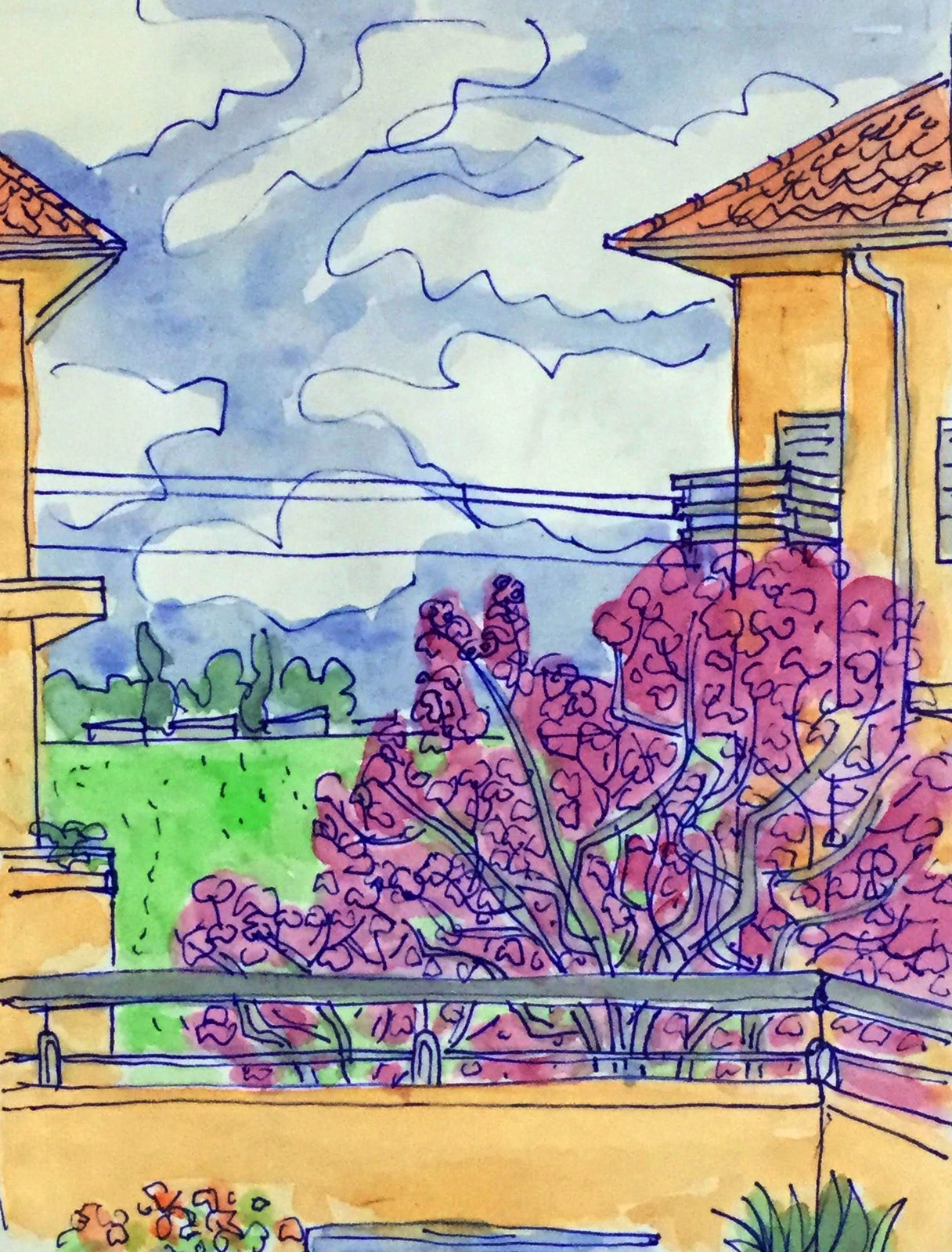The artwork is a detailed painting, possibly done with watercolor or magic markers, depicting a tranquil scene from what seems to be a balcony view. The sky in the background is a mix of purplish and bluish hues adorned with white fluffy clouds. The painting features two orange to brownish-orange colored houses with red roofs, spanning across the upper and lower left as well as the upper and lower right sides of the picture. Some of the houses feature rain spouts and electrical wires connecting them. Centrally located between the houses is a garden area with a tree line and a vibrant green grassy field. Prominently in the middle is a large bush with purple flowers or leaves, contributing to the floral display. At the bottom of the image, where the balcony rail with silver elements is visible, there are more flowers and plants. The balcony's railing appears to be made of metal, and potted plants or flowers can be seen lining its lower part.